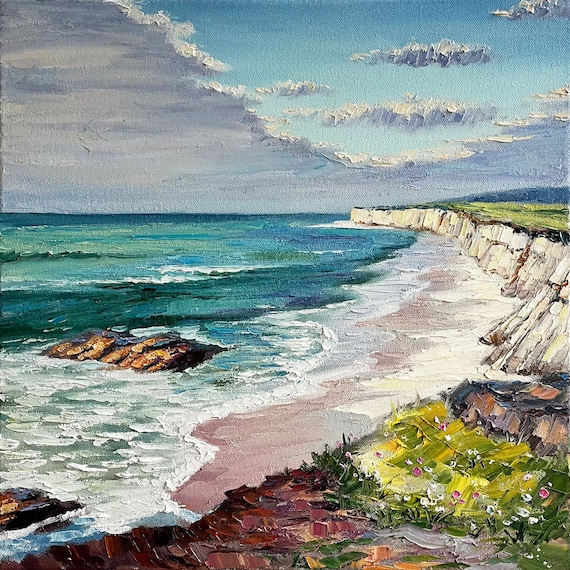The image depicts a vivid seascape painting, likely created with oil-based paints or watercolors, featuring a detailed ocean shoreline. The composition is rectangular, slightly taller than it is wide. A brilliant blue sky occupies the top third of the image, accentuated by a U-shaped cluster of clouds near the horizon and a few smaller clouds dispersed in the sky.

The left side of the image showcases a bluish-green ocean, with churning white foam cascading onto the shore. The shoreline itself varies in color, with darker sand where the water washes up and lighter, almost purple and gray hues closer to the ridge line. A reef or rock formation with additional rocks protruding from the water can be seen towards the left side of the image.

On the right side, a grassy land ridge rises slightly above the shoreline, adorned with white and pink flowers near its base. Amongst the green grass, the rock wall further enhances the natural beauty of the scene. The watercolor-like quality and the rich, vivid colors of the entire painting, including the meticulously detailed grass, flowers, and waves, contribute to the overall serene and picturesque ambiance.